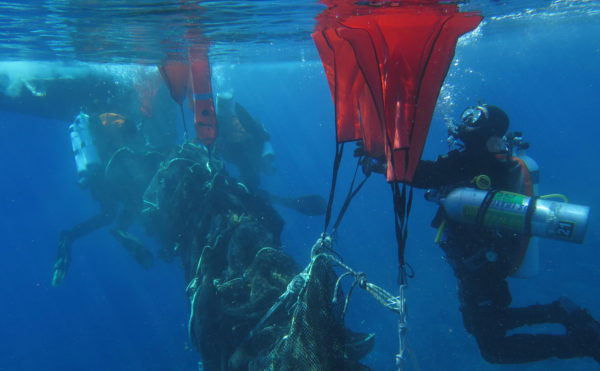This underwater photograph captures a dynamic scene of several scuba divers engaged in underwater tasks near the surface, with sunlight filtering through the water. On the right-hand side, a diver in full scuba gear with an air tank strapped to his side is seen with his arms outstretched, either tying or untying knots from red flotation devices. These devices, resembling parachutes or cones, are connected by straps to sea debris or netted objects, securing them in place just below the surface. In the background, the bottom of a boat looms, and more divers can be seen working amidst additional reddish-orange flotation devices, creating a coordinated effort that suggests a training or installation operation.